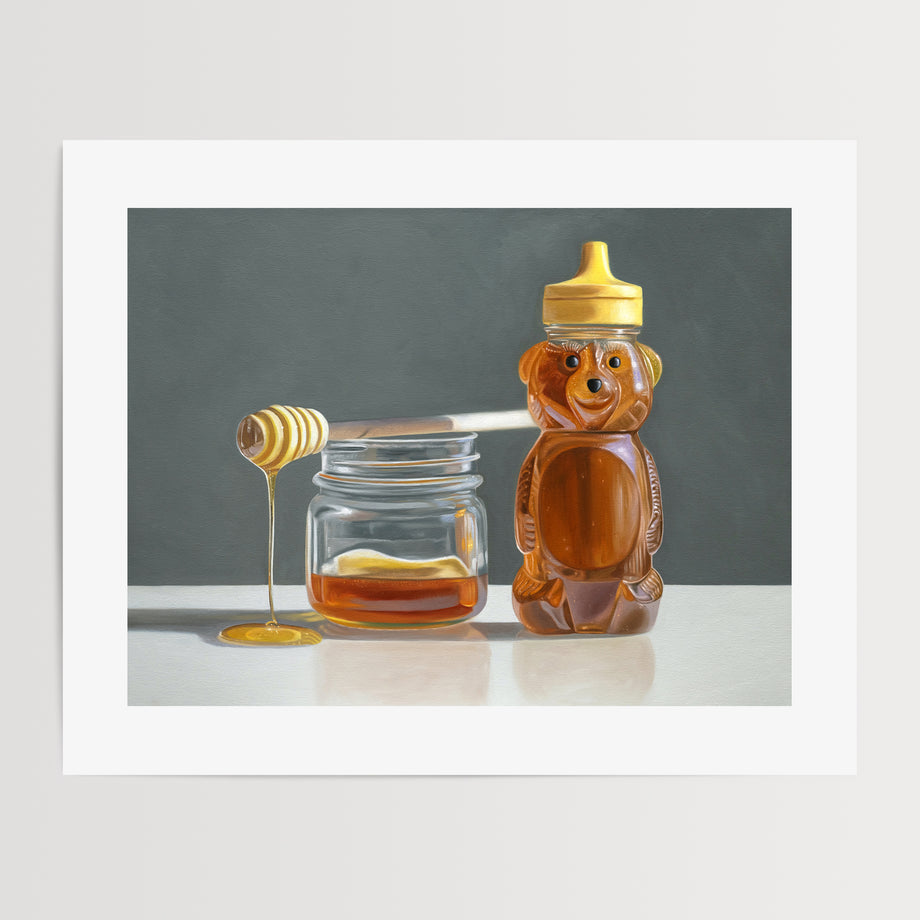This image showcases a vibrant hand-painted artwork displayed indoors on a white wall, framed with a white border. The painting depicts a bear-shaped honey container, filled to the brim with golden honey, with distinctive black eyes, nose, and a cheerful smile. The container has a yellow cap that pops open. To its right, there is a half-filled glass jar of honey, about the size of a baby food jar. Resting on top of this jar is a traditional honey dipper, with honey visibly dripping from it. The background of the painting is a soft, light grey. Both the countertop and wall in the photograph are grey, creating a cohesive and soothing backdrop.